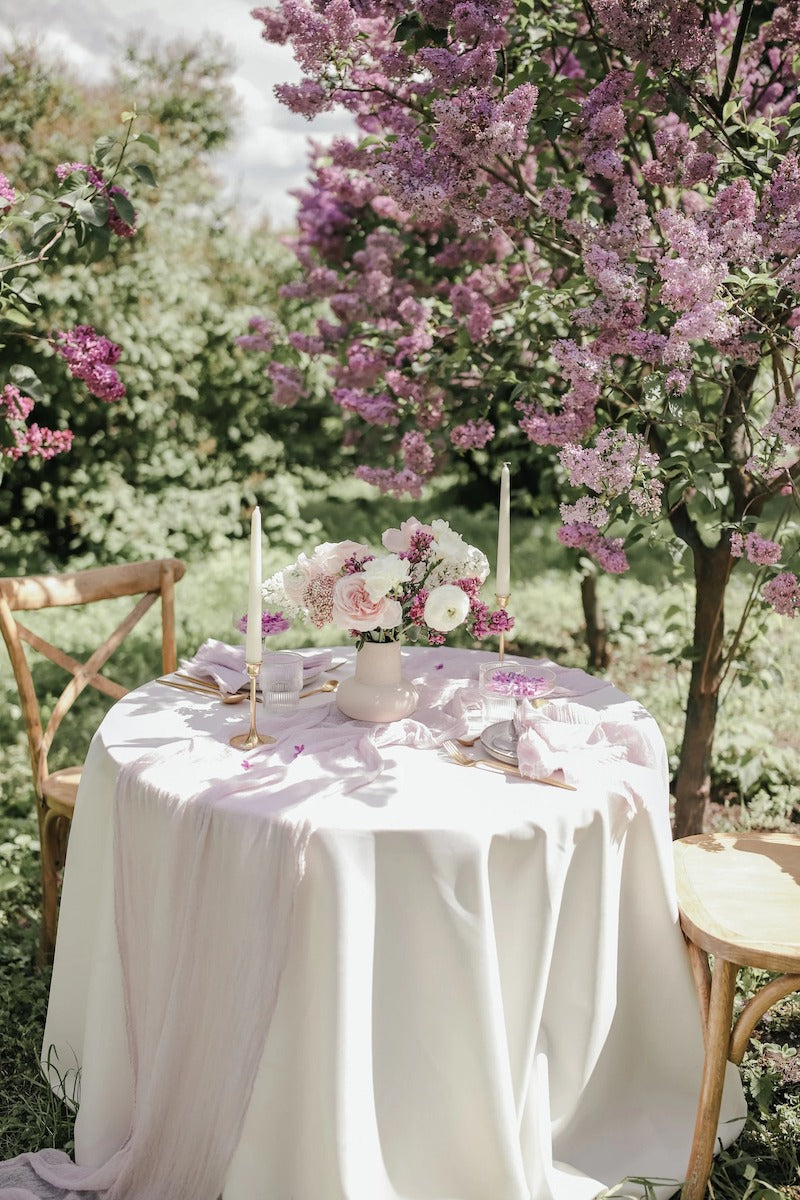The photograph captures a serene and beautifully set outdoor dining area bathed in sunlight. Central to the image is a round table draped in a flowing white tablecloth that puddles gently onto the grass. On the table, a white ceramic vase holds a delicate arrangement of white, pink, and lavender flowers, adding a touch of elegance. Flanking the vase are two gold candle holders with white tapered candles, suggesting a romantic setting. The table is meticulously arranged for two, complete with plates, gold utensils, and neatly folded napkins. Two wooden chairs with light finishes stand on either side of the table. In the backdrop, a lush garden unfolds with cherry trees in full pink blossom, lilac bushes pruned into tree forms, and a vibrant carpet of grass and ground plants. Sunlight filters through the trees, enhancing the image’s calm and inviting ambiance, although a cloudy sky hints at a gentle overcast above.